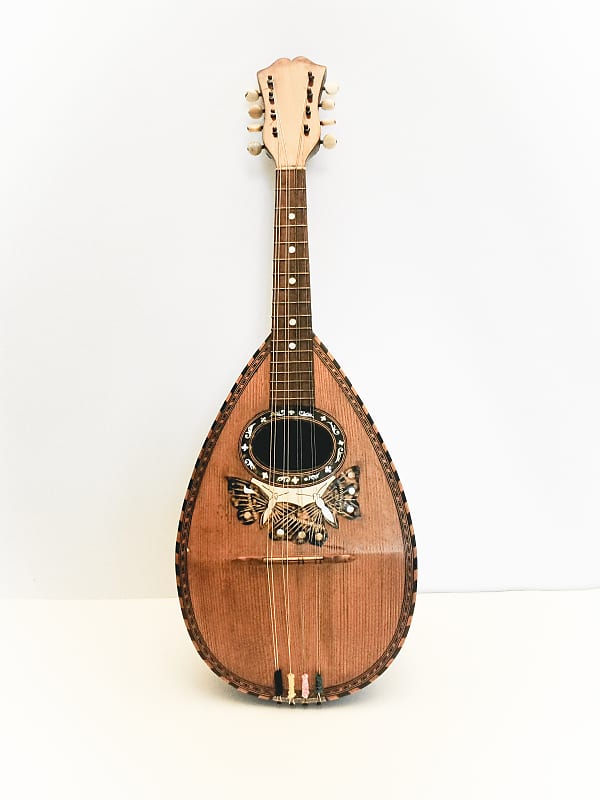The image depicts a wooden mandolin positioned against a grey wall with a very light grey floor beneath it, creating a nearly monochromatic background. The mandolin, a central focus, showcases a light brown, wooden body with ornate detailing. The instrument features a light wooden neck with cream tuning pegs arranged in two rows of four at the top. The main body includes a beautifully intricate design: two butterflies with black and white wings emerge from around the instrument's soundhole. The soundhole itself is surrounded by a decorative black and white border, enhancing the intricate aesthetic of the mandolin. The subtle detailing of the butterflies and the cream strings against the wooden backdrop highlights the craftsmanship and elegance of the instrument.